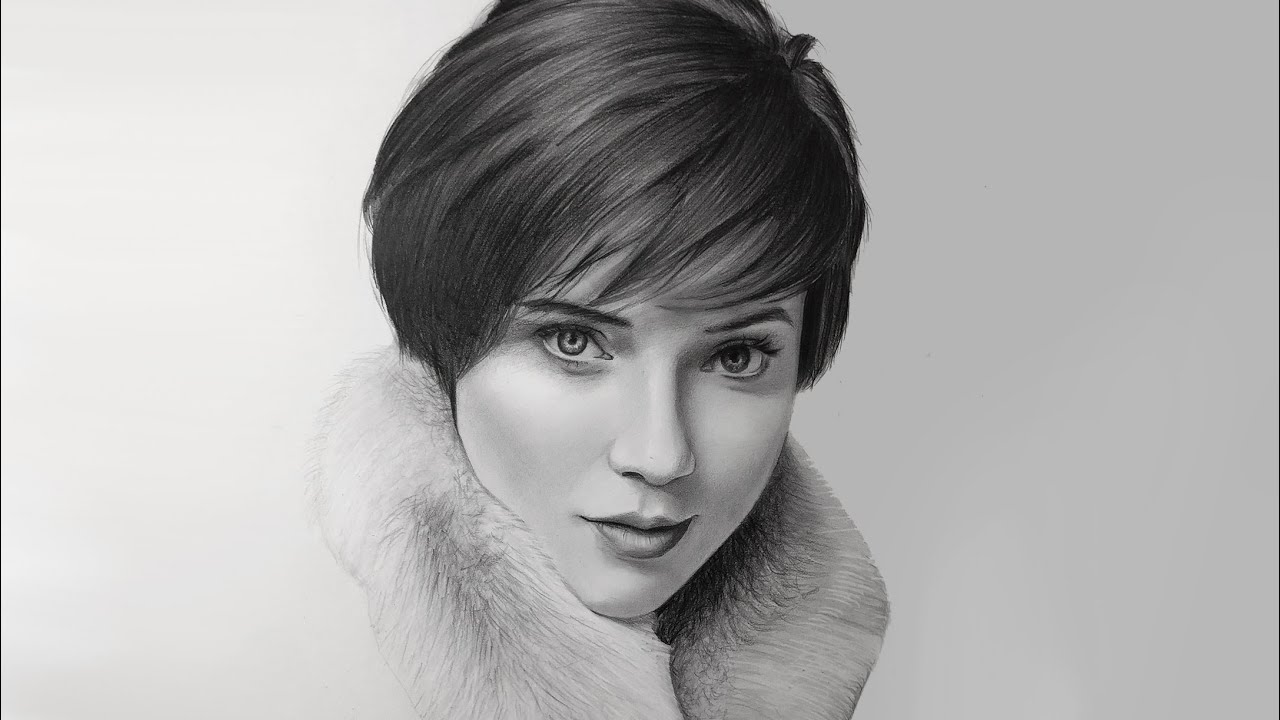This black and white pencil portrait features a detailed close-up of a white woman with a short, straight hairstyle that just reaches her ears, although her ears are not visible. She has larger, expressive eyes staring directly at the viewer, with her face slightly downturned. The woman wears a fur collar around her neck, which is drawn close to her chin, obscuring her neck and any other parts of her body. The background remains untouched by pencil, providing a stark contrast against the darker tones of the paper, which may appear grey due to shadows from photographing the illustration. Her hair is neatly combed to the side, and the meticulous detailing in the eyes, hair, and fur collar highlights the sketch's precision.